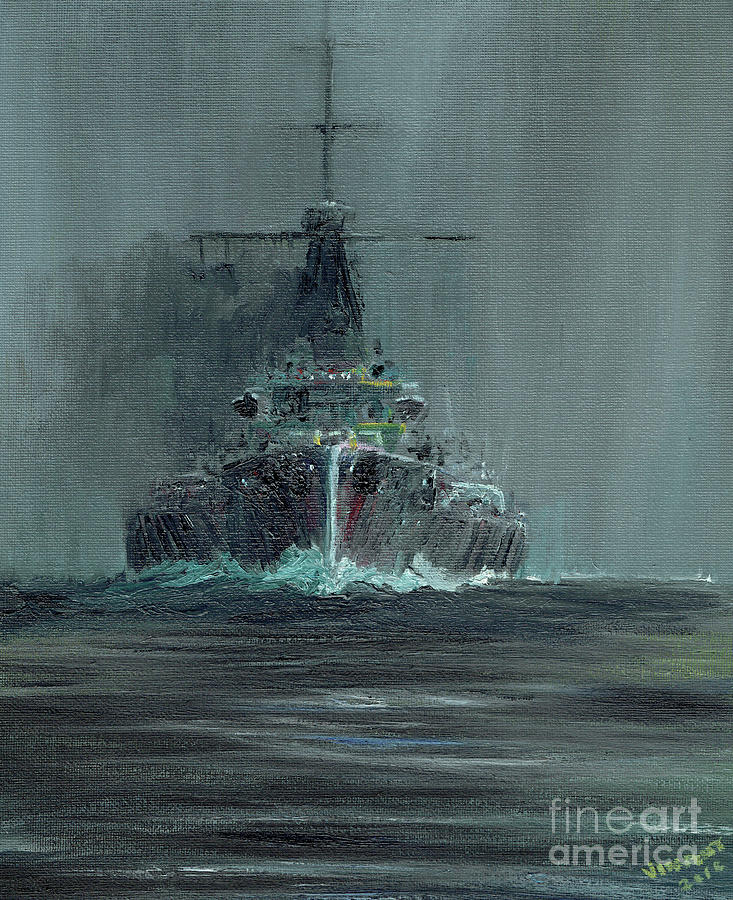This artwork, dated either 2016 or 2018, is a loosely painted and abstract oil painting, predominantly in dark and murky tones of gray, green, and blue. The scene captures a stormy night at sea, with a ship emerging hazily in the background, partially obscured by fog. The painting employs broad, indistinct strokes to depict the turbulent water smashing against the vessel, enhancing the chaotic and obscure nature of the environment, where the sky and sea blend into each other in various shades of dark gray and black. In the bottom right-hand corner, there is a visible watermark reading "Fine Art America," along with the artist's signature, which begins with a "V" but remains unreadable. The signature and year—2016 or 2018—are all that can be discerned from the inscription.